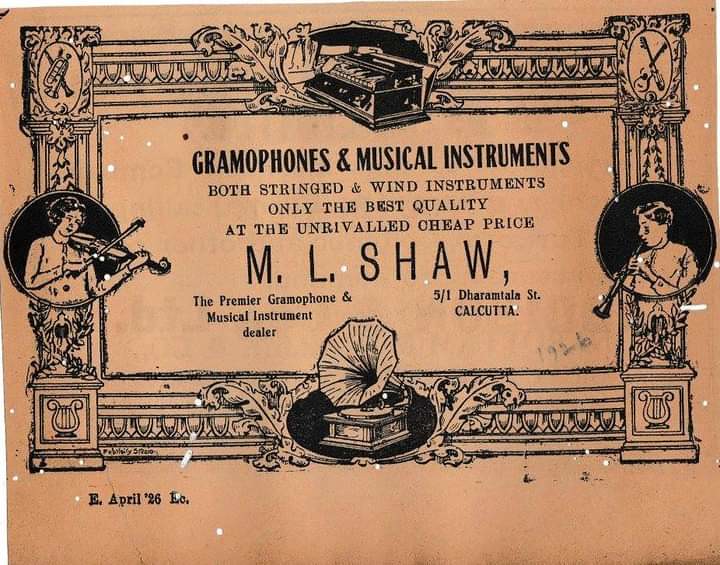This image appears to be a vintage advertisement from 1926, featuring elaborately detailed artwork and text. The advertisement, printed on faded beige paper with deep blue or black text, showcases ornate Romanesque borders with small illustrations in each corner. In the top-left corner, a woman plays a violin, while on the top-right, a man plays a flute. At the bottom corners, additional sketches depict musical scenes, including an old-fashioned phonograph. Central to the ad, bold text announces "Gramophones and Musical Instruments, both stringed and wind instruments, only the best quality at unrivaled cheap prices." The prominent name "M.L. Shaw," identified as the premier gramophone and musical instrument dealer, is displayed underneath, along with the address "5-1 Dharamtala Street, Calcutta." The ad also bears the penciled-in date "April 26, 1926," marking it as a relic from that year.